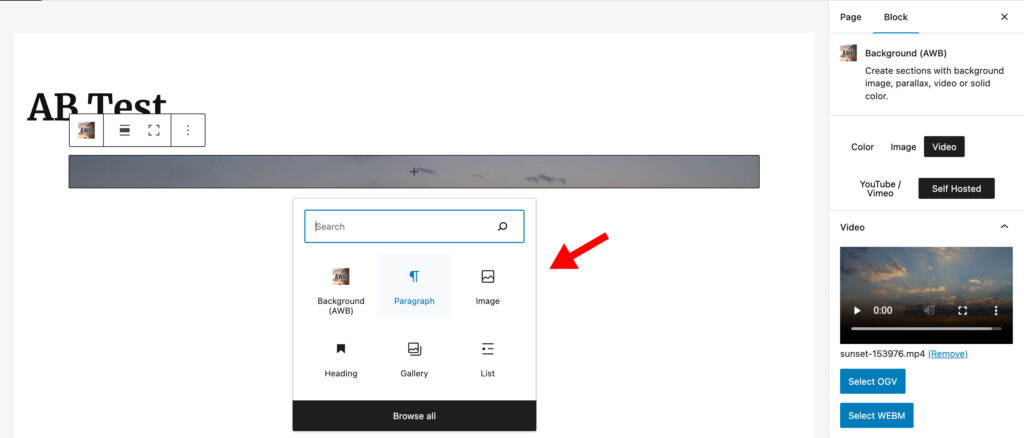This is a detailed description of a screenshot depicting a web application interface. The background is predominantly white. On the left side of the screen, we see a full webpage framed by off-white borders at the top, left, and right edges. In the upper-left corner of the webpage, there is the text "A/B Test" displayed in black font. Superimposed above this text are four small squares, each containing a faint icon. The icon on the far right of these squares consists of three vertical black dots.

Below this section, there is a gray bar stretching across the width of the webpage. Directly beneath the gray bar is a black-outlined square set against the white background. This square contains a search field at the top. Inside the search field, the word "Searching" is written in black font, accompanied by a black magnifying glass icon positioned on the far right of the field.

Further down, there are two rows of selectable options within the outlined square. The first row features the options "Background," "Paragraph," and "Image." The second row includes "Heading," "Gallery," and "List." Notably, a red arrow, presumably added via Photoshop, is pointing towards the "Image" option.